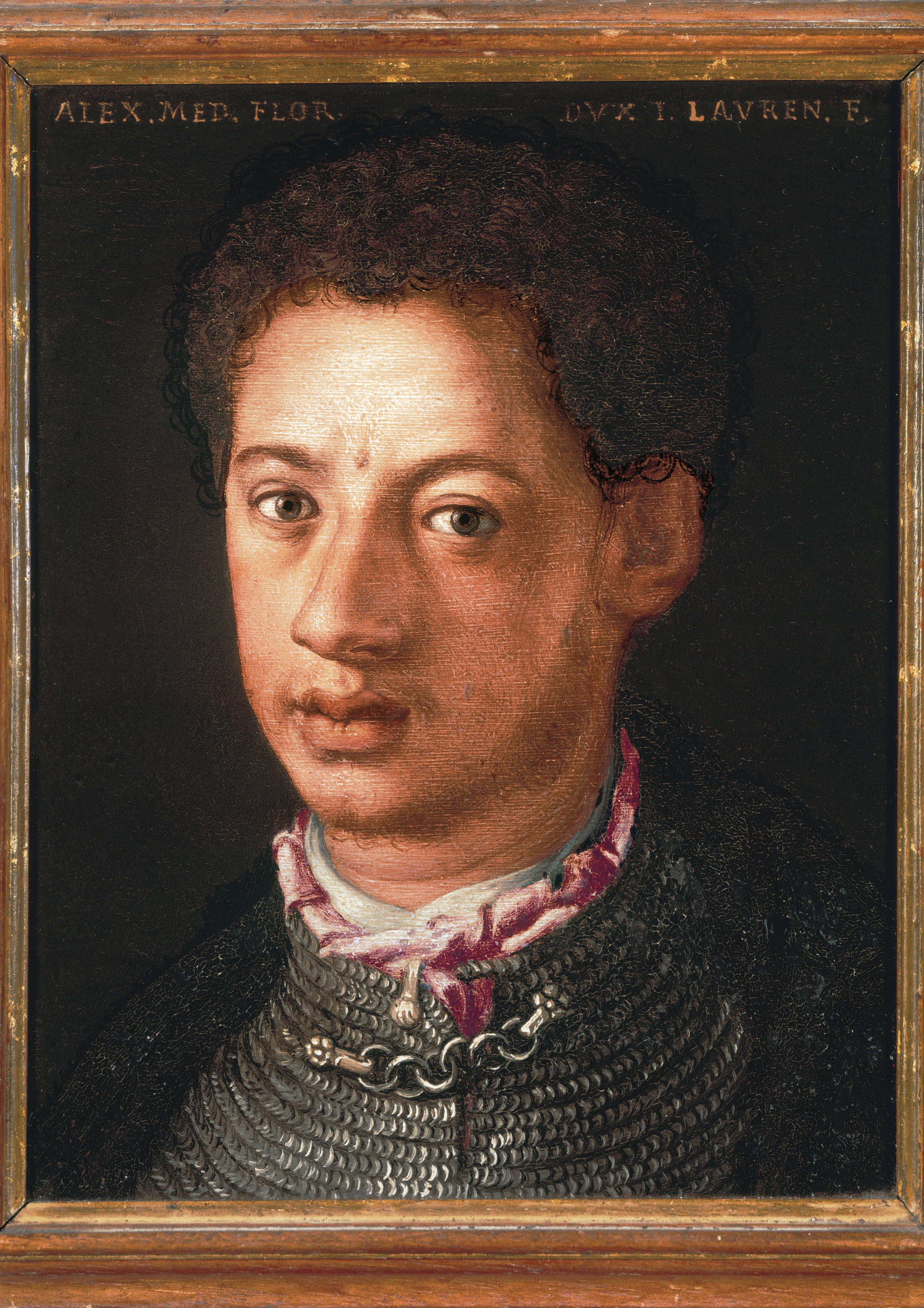The image is a painted portrait of Alex Medfloor, created by an artist named T. Leverne F. The portrait features a man of light complexion, possibly African American or Hispanic, with curly hair framing his forehead. His eyes are a striking hazel or light brown, giving him a piercing gaze that looks directly at the viewer. His expression is neutral, neither happy nor sad, but rather content and composed.

Alex Medfloor is attired in what appears to be a historical costume, with a hint of armor or chain mail beneath a high-necked garment, likely clasped together with a steel chain. Over this, he wears an overcoat that is secured at the chest. Around his neck, various thin scarves or ribbons of red and white colors are tucked in, adding a distinct touch to his ensemble. The background of the portrait is a dark black or gray, which makes the subject stand out prominently. The portrait is framed in wood, adding to the overall antique and slightly haunting feel of the image.